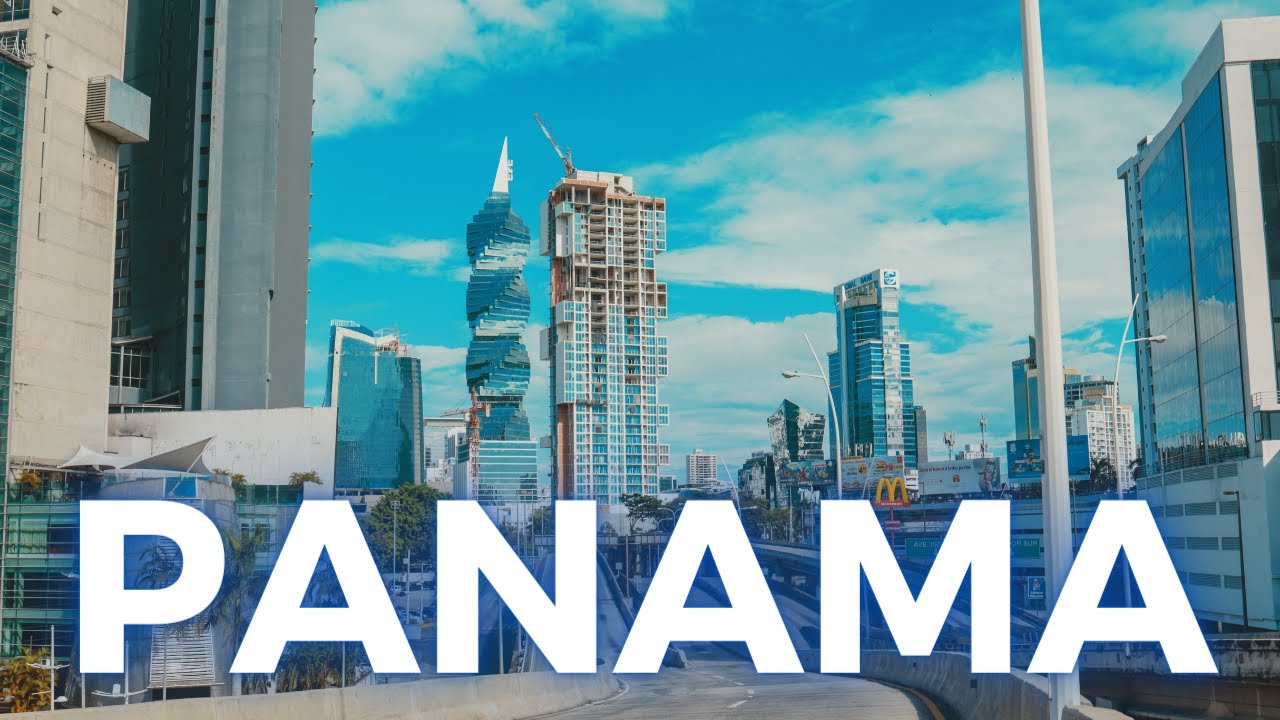The image prominently features the word "PANAMA" in bold, white, capital letters with a bluish glow surrounding them. The background showcases the bustling skyline of Panama City, with numerous high-rise buildings and skyscrapers. On the left, there are residential apartment buildings, while to the center and right, there are modern commercial structures with shiny blue glass facades. One distinctive skyscraper stands out with its twisted, spiraling design, capped by a white point.

At the bottom right of the image, a McDonald's sign is visible among several billboards and streetlamps. Further into the background, behind the glowing letters, you can see highways interspersed with patches of greenery. The sky above is a vibrant blue, dotted with scattered white clouds, adding to the dynamic and vibrant atmosphere of the cityscape. Another notable skyscraper in the backdrop has an expansive blue facade, contributing to the modern and sleek aesthetic of the panorama.